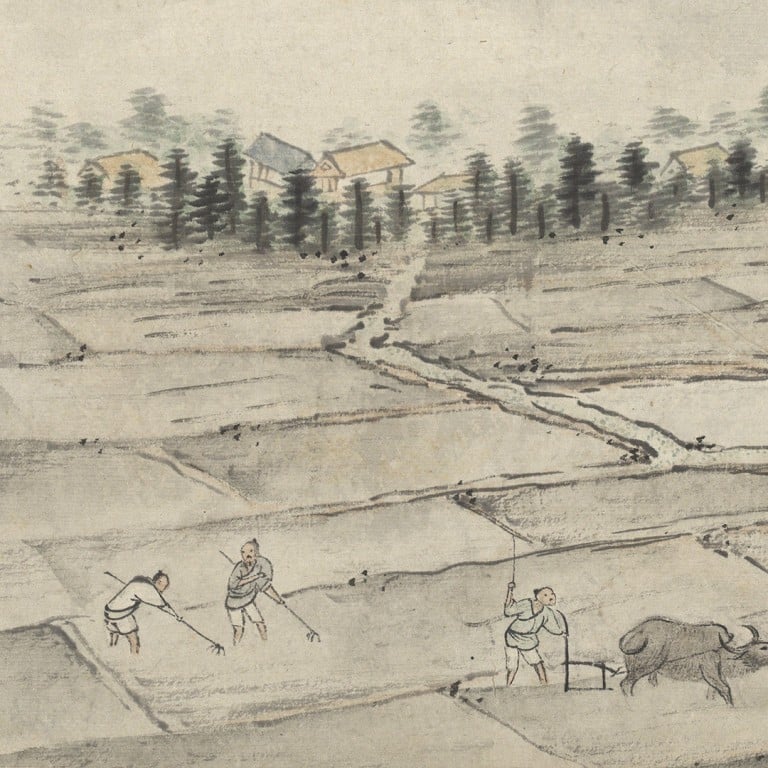This is a simple yet evocative pencil drawing done primarily in black, white, gray, and muted charcoal tones, with accents of beige and faded colors. The scene is depicted in a Southeast Asian style. In the foreground, a vast farm field stretches towards the background, resembling a traditional rice field. Three men, seemingly Asian farmers dressed in gray tunics and white pants, are engaged in labor. To the right, one farmer guides a gray ox or water buffalo, which is harnessed to a simple, old-fashioned wooden plow. This farmer holds a whip in his hand. On the left side, two other farmers work with hoes or rakes; one is bent over raking the ground, while the other stands upright, looking back. Further back, a long, winding path leads through the field towards a line of undetailed pine trees. Behind these trees, nestled in the background, are small huts or sheds. These modest structures have roofs or walls that are a pale beige or faded yellow, with one sporting a faded blue roof. The sky above is a mix of beige and gray tones. Overall, the composition is delicate, with a focus on traditional agricultural life in a serene, muted landscape.